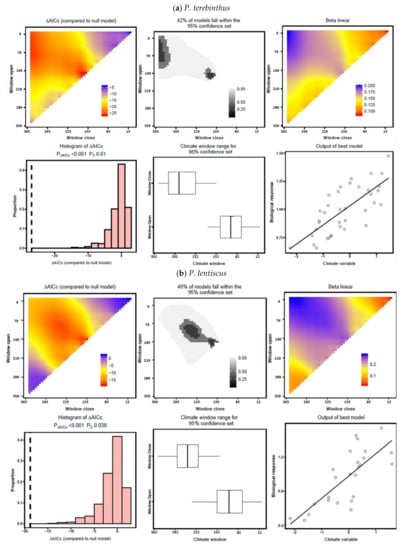The image comprises 12 distinct graphs and schematics arranged in a 4x3 grid. The text above and below each graph is small and difficult to read. The first and third rows feature thermal diagrams on the leftmost and rightmost graphs, showing triangles with gradients of colors including purple, pink, red, orange, yellow, and white. These graphs have legends that depict a color spectrum from purple to yellow to orange to red, illustrating varying intensities or data points. In the middle of these rows are grayscale plots, transitioning from white to black, with clusters of gray and black splotches suggesting focused data points or specific areas of interest.

The second and fourth rows share a similar structure: starting with bar graphs where the rectangles increase in height progressively, a graph with two squares connected by a horizontal line, and a scatter plot featuring a line with dots densely clustered along it, illustrating some form of correlation or data trend. Each graph in these rows appears detailed with labeling on the axes, although the text is too small to decipher. Overall, the image provides a complex array of graphical information that combines thermal visuals with varied data presentations in grayscale and bar formats.